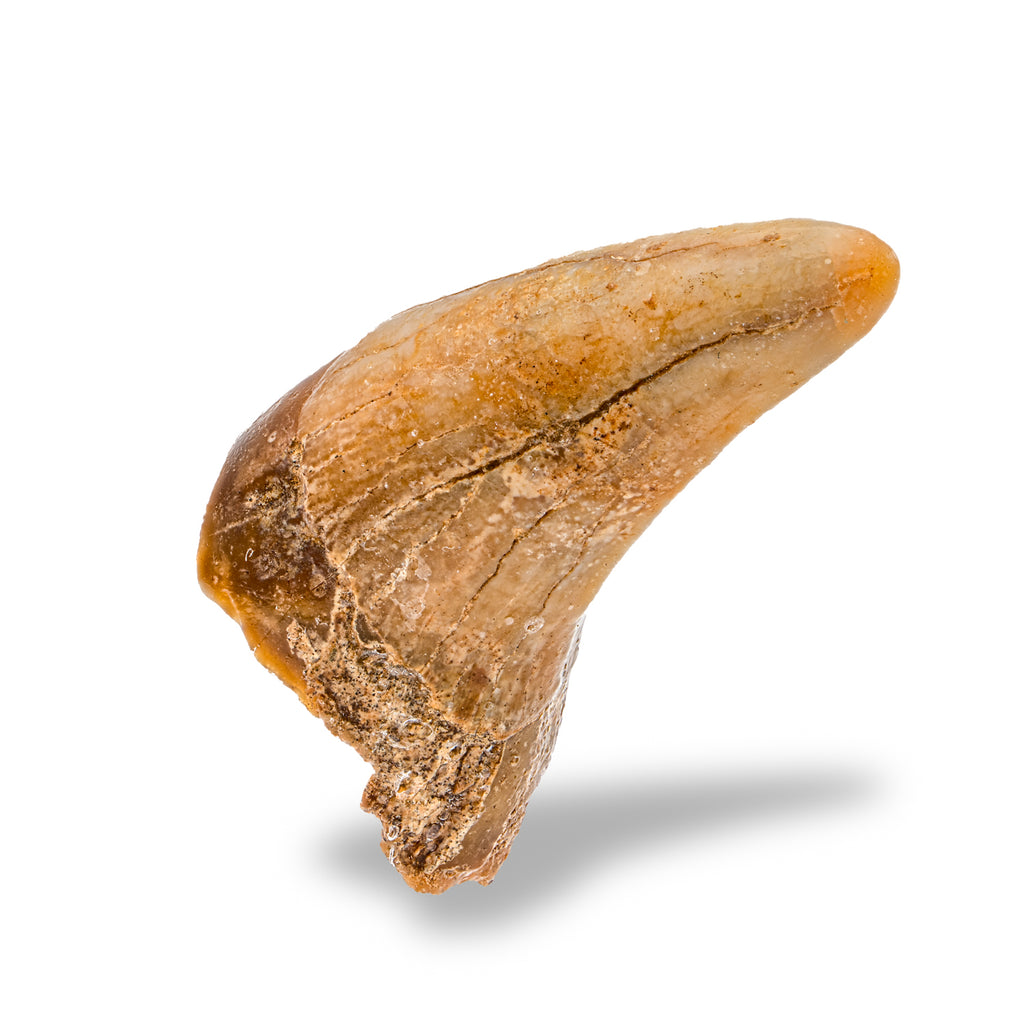The image is a close-up of an ancient, discolored tooth set against a plain white background. The tooth, appearing to belong to a large predator, displays multiple shades of brown and orange, with the base exhibiting a darker brown hue while the tip lightens to a beige color. The pointed end of the tooth is oriented towards the top right, creating an L-shape, with some areas showing clear signs of age through cracks, fissures, and decay. Calcium buildup is visible near the jagged base, adding to its ancient appearance. The detailed image highlights the tooth's intricate textures and aged characteristics, making it look like a fossilized, significant piece of paleontological interest.